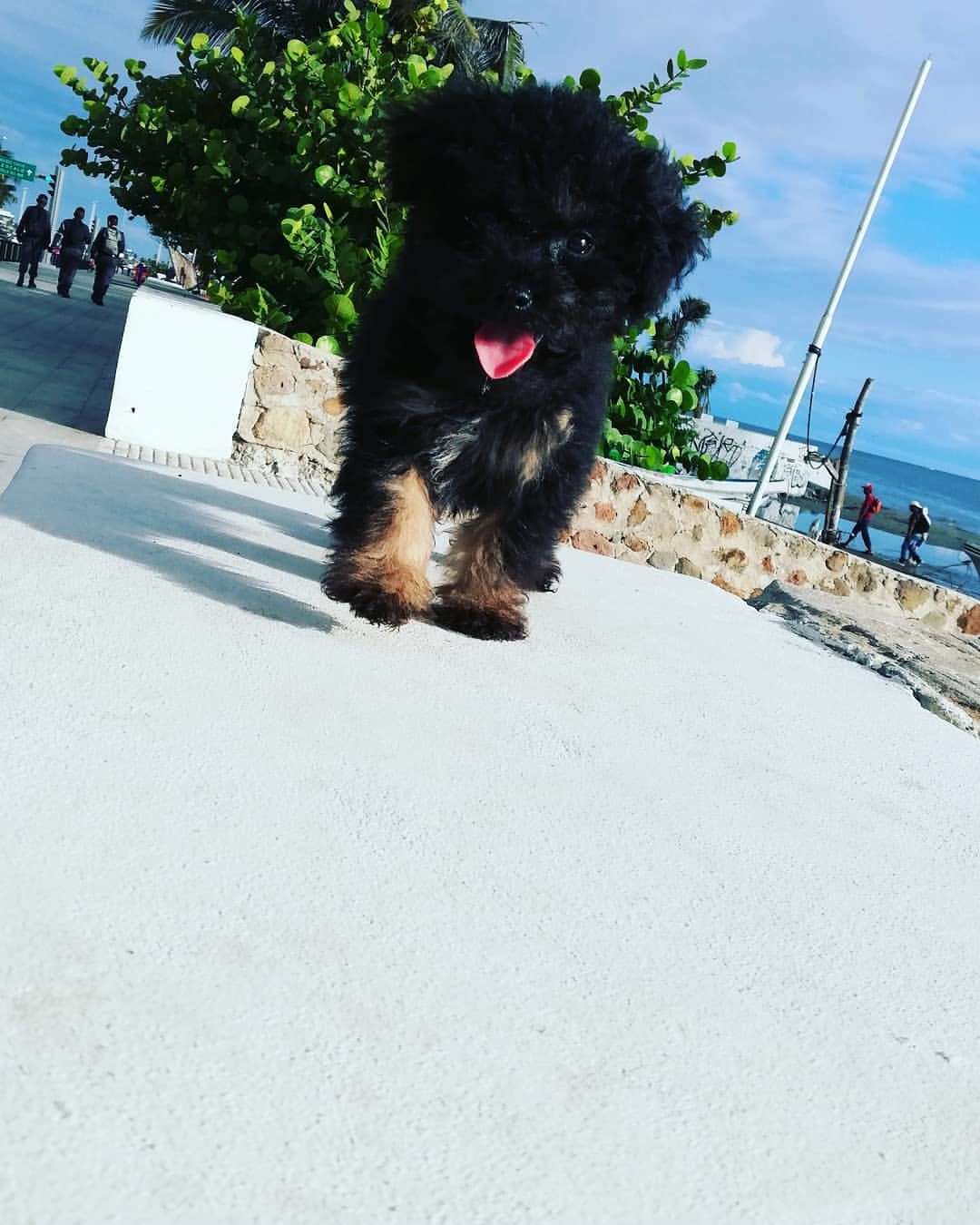In this detailed outdoor scene, a small, fluffy black dog with light brown paws and a small white patch on its chest is captured running directly towards the camera, its pink tongue playfully extended. The dog is centrally positioned on a stone-tiled walkway, which lies adjacent to a rocky area to the left. Just behind the dog, a low stone wall stands firmly, topped by lush greenery consisting of various trees, including a notable palm tree reaching towards the sky at the top of the image.

In the background, the serene blue ocean stretches out, accompanied by stretches of sandy beach where three people can be seen walking away from the camera. Above them, a street sign gently sways. Further into the distance, a boat can be spotted on the water. The sky above is dotted with soft clouds, adding a tranquil touch to this midday scene. The overall color palette of the image includes hues of blue, white, gray, green, black, brown, and tan, painting a vivid picture of a lively yet peaceful outdoor environment.